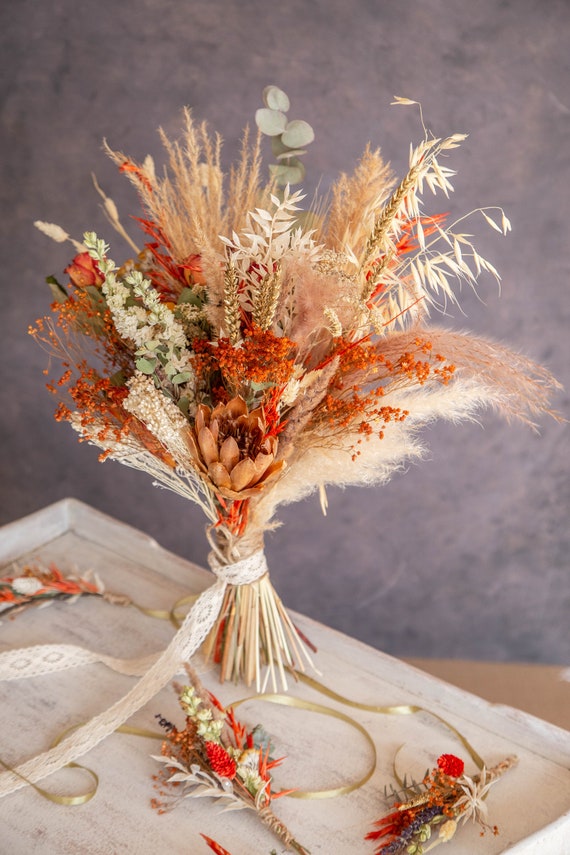The image depicts a detailed and intricate bouquet of dried flowers and native plants, artfully arranged on a light bleached wood tray. The bouquet features a variety of natural elements, including tall wheat grasses, tufty wild grasses, foxtail-like grass, and small sprigs of dried baby's breath. It includes an array of colors like earthy beiges, tans, oranges, deep reds, and pale greens, complemented by small peach-colored and tiny dried red flowers, as well as some delicate sage green sprigs. The bouquet is elegantly tied with a long off-white lace ribbon, which drapes gracefully off to the side and around the tray. Scattered around the arrangement on the tray are additional loose pieces of dried flowers and plants, enhancing the rustic charm of the composition. The background features a subtle, speckled light gray wall with a marbled, mauve, and rose-colored effect, creating a soft contrast to the earthy tones of the bouquet and the tray.